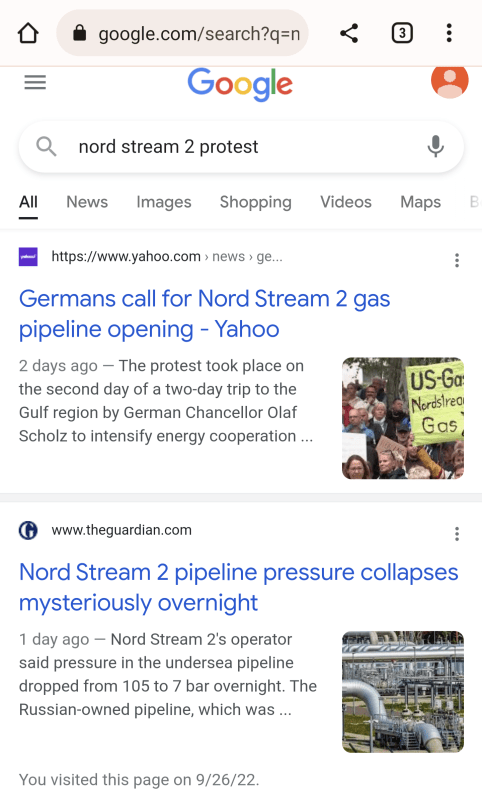This is a detailed screenshot of Google search results. At the top of the screenshot, the iconic Google logo is displayed prominently. To the right of the logo, the default Google profile image appears, showcasing a stick figure against an orange background.

The search query entered in the Google search bar reads "Nord Stream 2 Protests." Directly below the search bar, various search result categories are available: All, News, Images, Shopping, Videos, Maps, and an additional, slightly cut-off tab. The current tab selected is "All."

The first search result is from Yahoo and is titled "Germans call for a Nord Stream 2 Gas Pipeline opening." It was posted two days ago. The snippet below the title describes the protest as occurring on the second day of German Chancellor Olaf Scholz's trip to the Gulf region, aimed at strengthening energy cooperation. Accompanying this result is an image of a protest on the right.

The second search result comes from theguardian.com with the headline "Nord Stream 2 Pipeline Pressure Collapses Mysteriously Overnight," published one day ago. The snippet informs that the operator of Nord Stream 2 reported a significant drop in pressure within the Idris Sea Pipeline, from 105 to 7 bar overnight. The sentence trails off with “which was...” suggesting further information is available by following the link. To the right of this result is an image of a pipeline.

Underneath the second result, there's a note stating, "You visited this page on 9-26-22."

The photo depicts the search results in Google's default light mode, providing a clear and easy-to-read layout of the information.